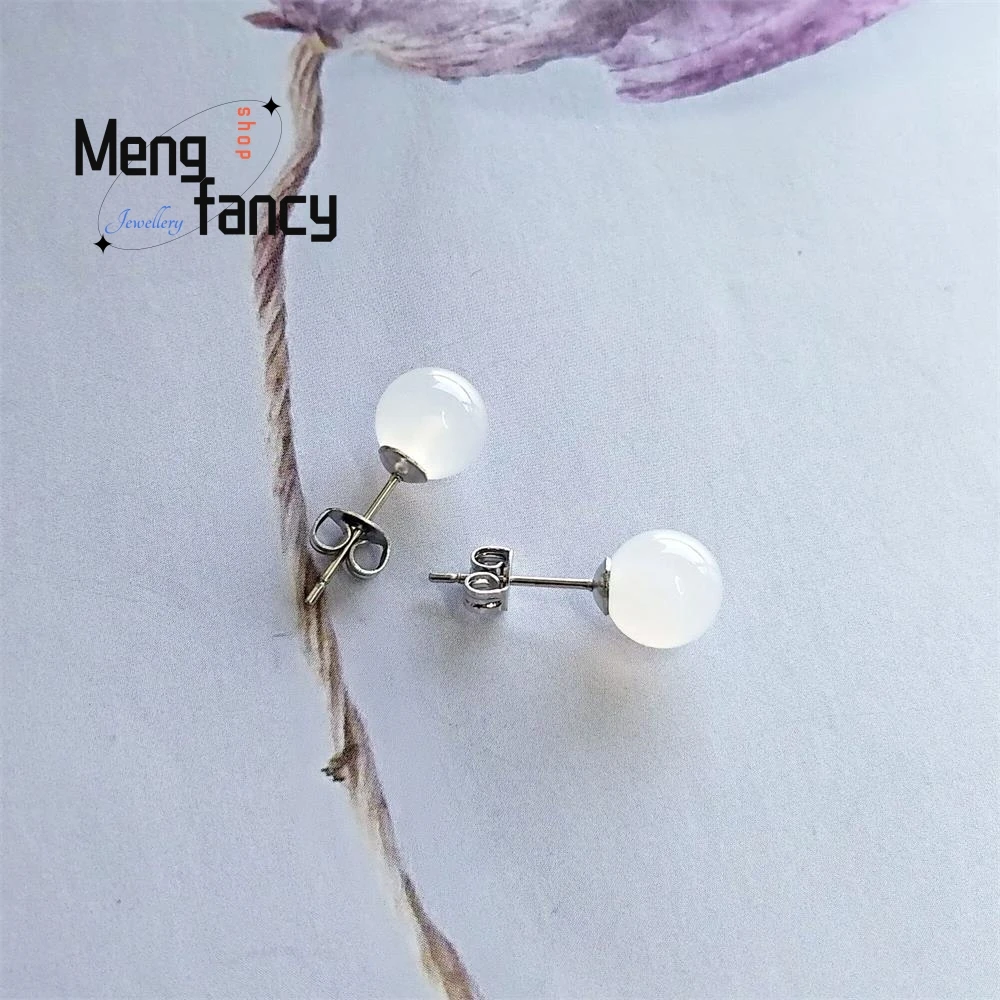The image showcases a pair of spherical, translucent white earrings resting on a silver base. They are arranged on a paper surface adorned with a subtle, partially visible design, potentially featuring a faint purplish-gray hue. Alongside the earrings runs a white string, which appears to connect to a small, possibly painted, purple flower or design near the top of the image. In the top left corner, a logo for "Meng Fancy Shop Jewelry" is prominently displayed within an oval frame, embellished with sparkles at the top right and bottom left. The logo features black text for "Meng" and "Fancy," vertically oriented orange lettering for "Shop," and horizontally placed blue text for "Jewelry." The overall composition suggests this is an advertisement for Meng Fancy Shop Jewelry, highlighting their elegant earring offerings.